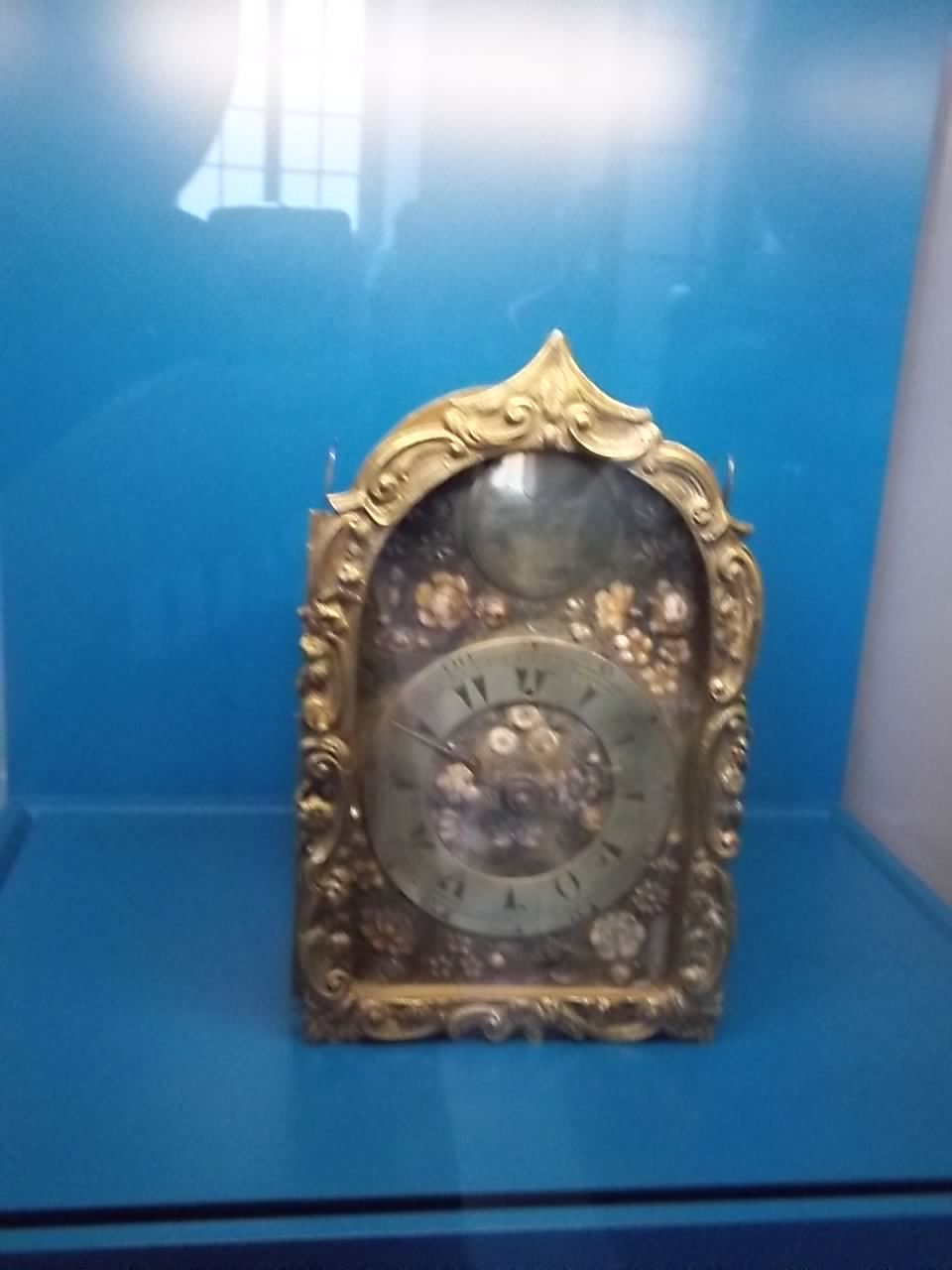This is a color photograph featuring a display case with reflective glass. The reflections in the glass include a person holding up a cell phone, likely the photographer. Inside the display case, there is an ornate clock with an intricate golden casing. The clock face is visible, with black icons indicating the numbers instead of traditional numerals. The clock casing also appears to house decorative floral elements, though the exact details are unclear due to the photo's slight blur. The interior of the display case, including the background and floor, is a light blue color, adding a subtle contrast to the golden hue of the clock.